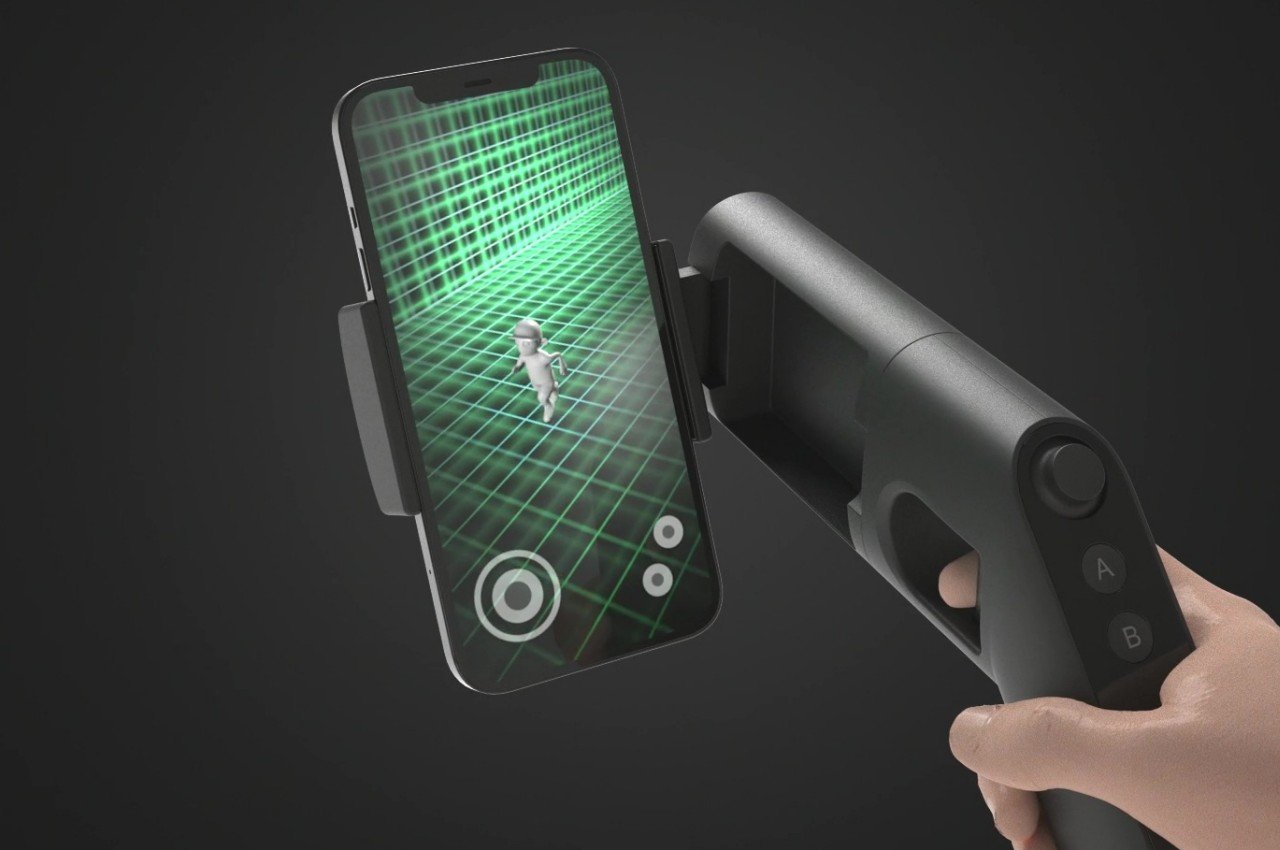The image depicts a black plastic gun-shaped controller with a trigger and multiple buttons, including labeled A and B buttons, designed to be used with a smartphone for gaming. The smartphone fits into a designated slot on the controller, which attaches securely around its edges. The scene on the smartphone shows a white, human-like figure navigating through a green and black plaid room or alcove, suggesting the setting of a shooting game. The background of the overall image is dark, emphasizing the white hand holding the controller coming from the bottom right corner. The detailed grip of the hand showcases the placement of fingers around the different buttons and trigger, indicating the controller's functionality for interactive gameplay.